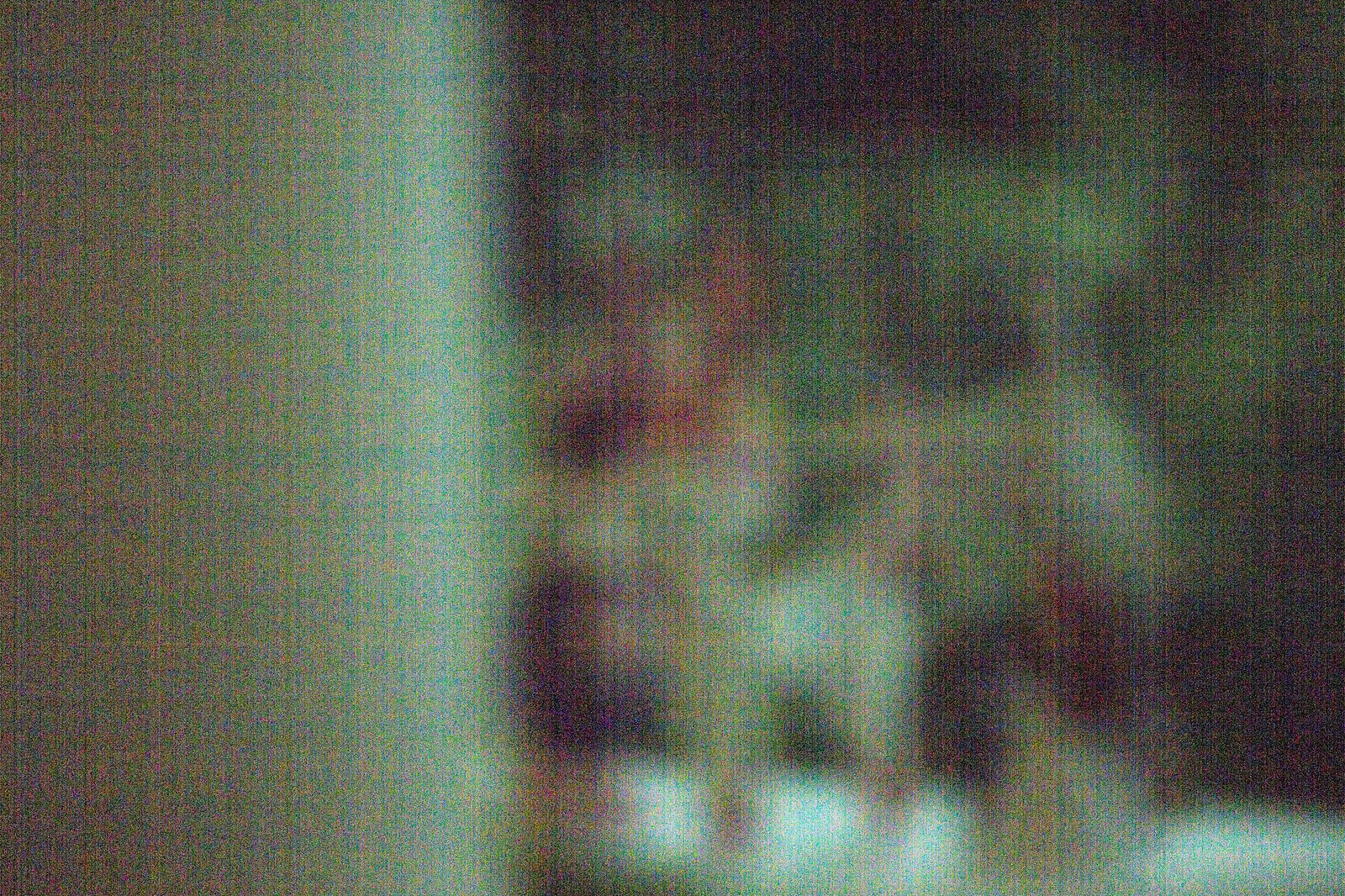The image is a blurry, grainy, and pixelated photograph that is difficult to decipher due to its highly distorted and staticky texture. It resembles a grid-like pattern with streaky lines running vertically and horizontally. The left side of the image features dull tan and light brown colors transitioning into white, while the right side showcases darker areas with black and gray tones, interspersed with lighter spots. Centrally, there's a patch of red, and various other colors, including green, dark gray, blue, pink, and yellow, can be observed throughout the image. The pixelation is so pronounced that individual pixels are visible, contributing to the overall impression of a staticky TV screen. Amidst the dark patches on the right, some interpreters perceive indistinct shapes that suggest the outline of a dog or even the close-up of a human face, although the extreme blurriness makes it impossible to definitively identify these forms. White spots also appear, especially towards the bottom right.